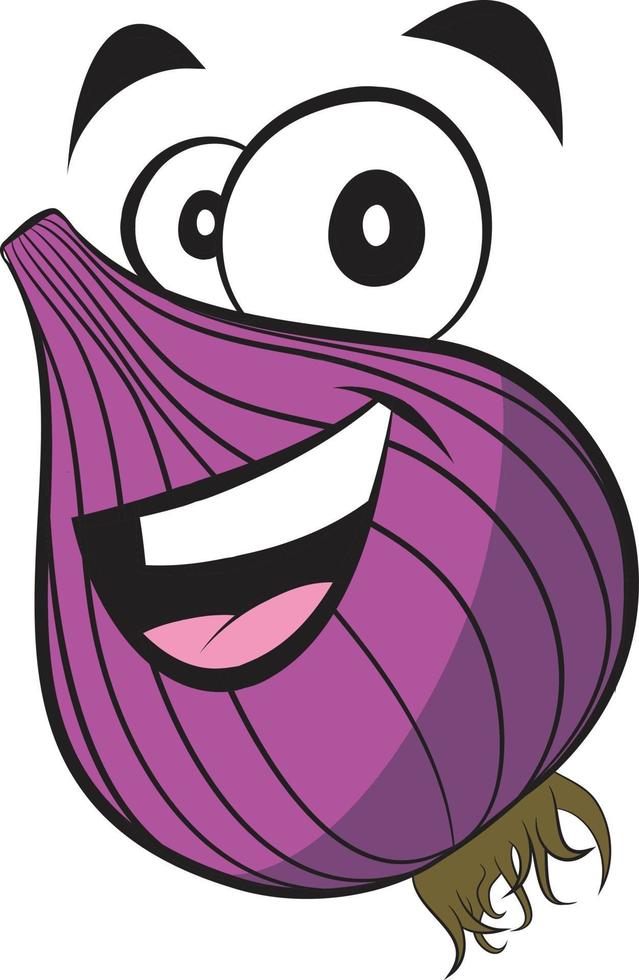The image is a detailed digital pen and ink representation of a cartoon character created from a red onion. The onion is depicted in varying shades of purple, highlighting its identity as a red onion. It has a pair of large, white eyes with black centers and expressive black eyebrows, positioned above the onion. The facial expression portrays a look of surprise or laughter. The cartoon character features an open mouth with visible top teeth and a pink tongue. The bottom part of the onion has solid brown coloring, resembling a beard formed by the exposed roots. While the onion's stems suggest a neck-like structure, a subtle light source illuminates the front of the face, creating a brighter appearance and casting shadows around the "chin" and sides, adding depth to the character. This imaginative artwork uses an onion to creatively form a humorous and lively cartoon figure.